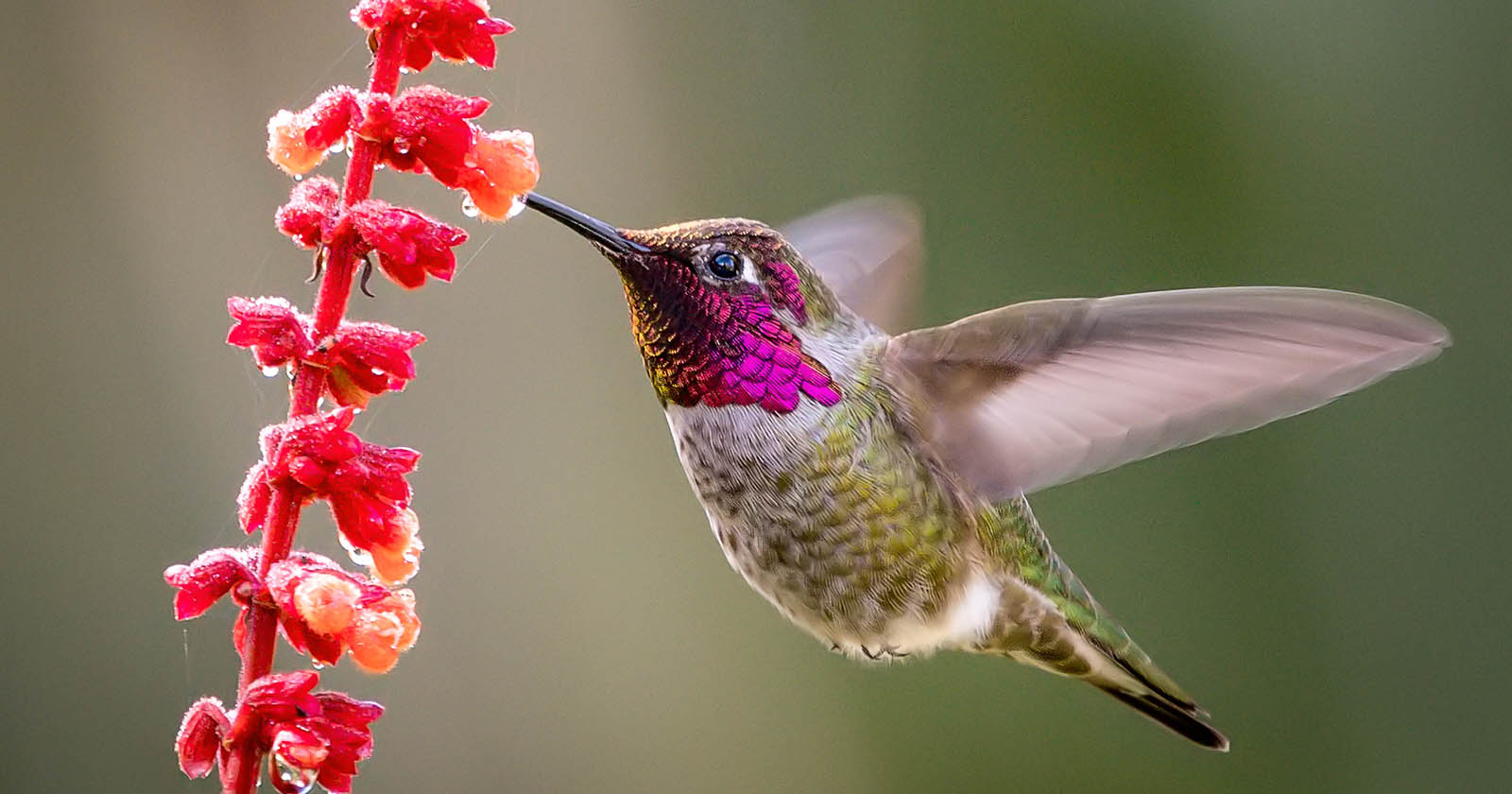In an extremely high-definition close-up wildlife photograph, a fascinating scene is captured featuring a hummingbird mid-air, drinking nectar from a vibrant coral-colored salvia flower. The flower, presenting a red stem with tubular blossoms, creates a colorful focal point on the left side of the image. The bird, potentially a western hummingbird rather than a ruby-throated variety, showcases a striking magenta patch of feathers around and under its eye, a greenish throat, and a white and green belly. Intricate details can be observed, from its black-tipped beak immersed in the flower's tubular blooms to its seemingly translucent wings frozen in motion against a blurred green background. This professional quality photograph, akin to those featured in National Geographic or Smithsonian, emphasizes the exquisite colors, fine feather details, and precise nature depiction, making the overall imagery both dynamic and captivating.